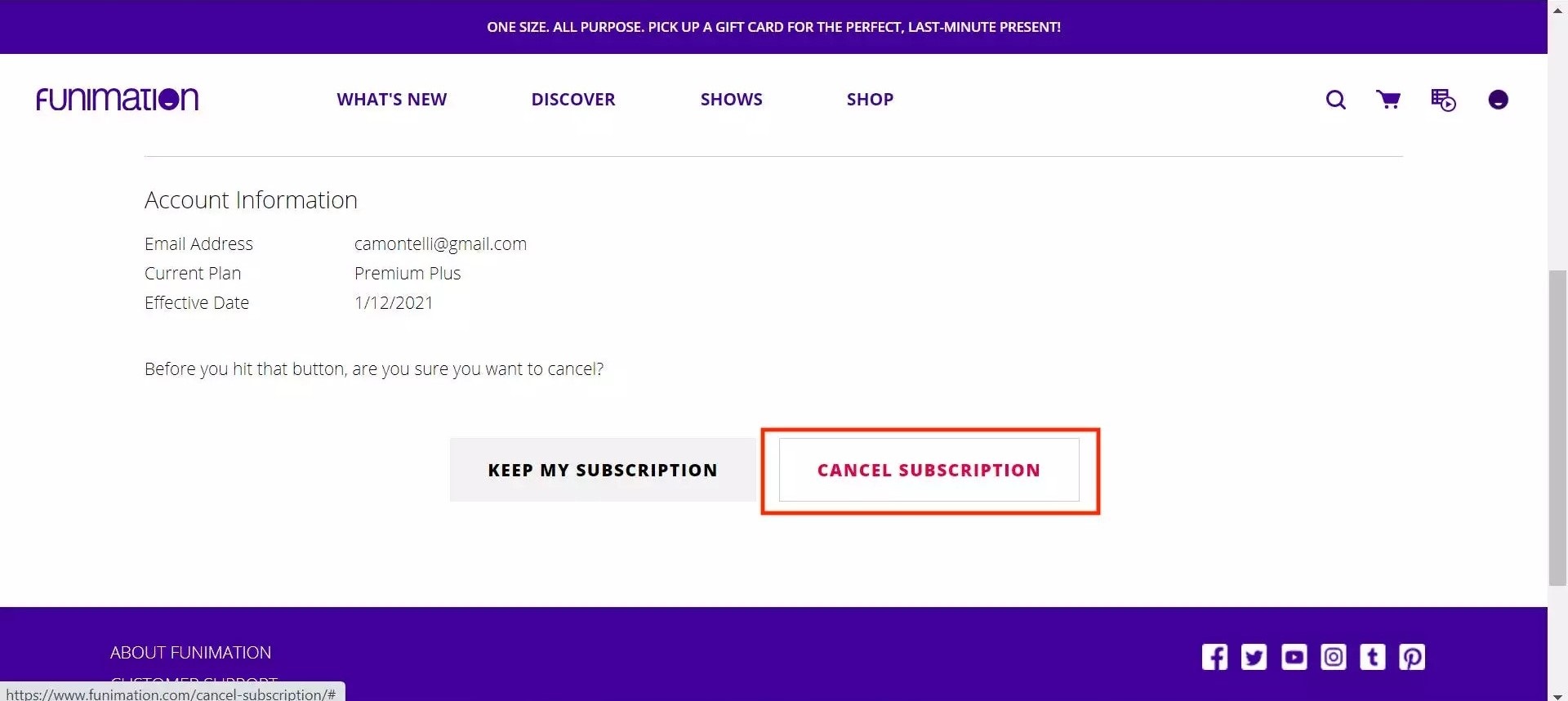The image depicts a user interface from a webpage. At the very top of the page is a narrow, deep purple rectangular banner. Beneath this, there is a slightly wider purple rectangular section at the bottom of the main interface. 

On the right side of the bottom purple section are several social media icons: Facebook, Twitter, Pinterest (represented by a 'P'), an icon resembling a 'T', a camera icon, and one featuring a square within a square.

Inside the top purple rectangle, the header features navigation words in purple: "Funimation", "What's New", "Discover", "Shows", "Shop", followed by a search icon, a cart icon, an icon with a square and a circle attached to its bottom right corner, and another icon resembling a mouth, with a small space not covered in purple. A light line is drawn beneath these words.

Below the header, the page content is organized into two columns. At the top of this section, it reads "Account Information." The first column lists "Email Address," "Current Plan," and "Effective Date." The second column provides the corresponding details: an email address, "Premium Plus Plan," and an effective date of "1-12-2021."

Under this information, there is a prompt: "Before you hit that button, are you sure you want to cancel?" To the right of this prompt are two buttons arranged horizontally. The first button, a gray rectangle, is labeled "Keep My Subscription." Next to it is another gray rectangle partially overlapped by a red rectangle, forming a combined button. The red portion of this button is labeled "Cancel Subscription" in red letters.